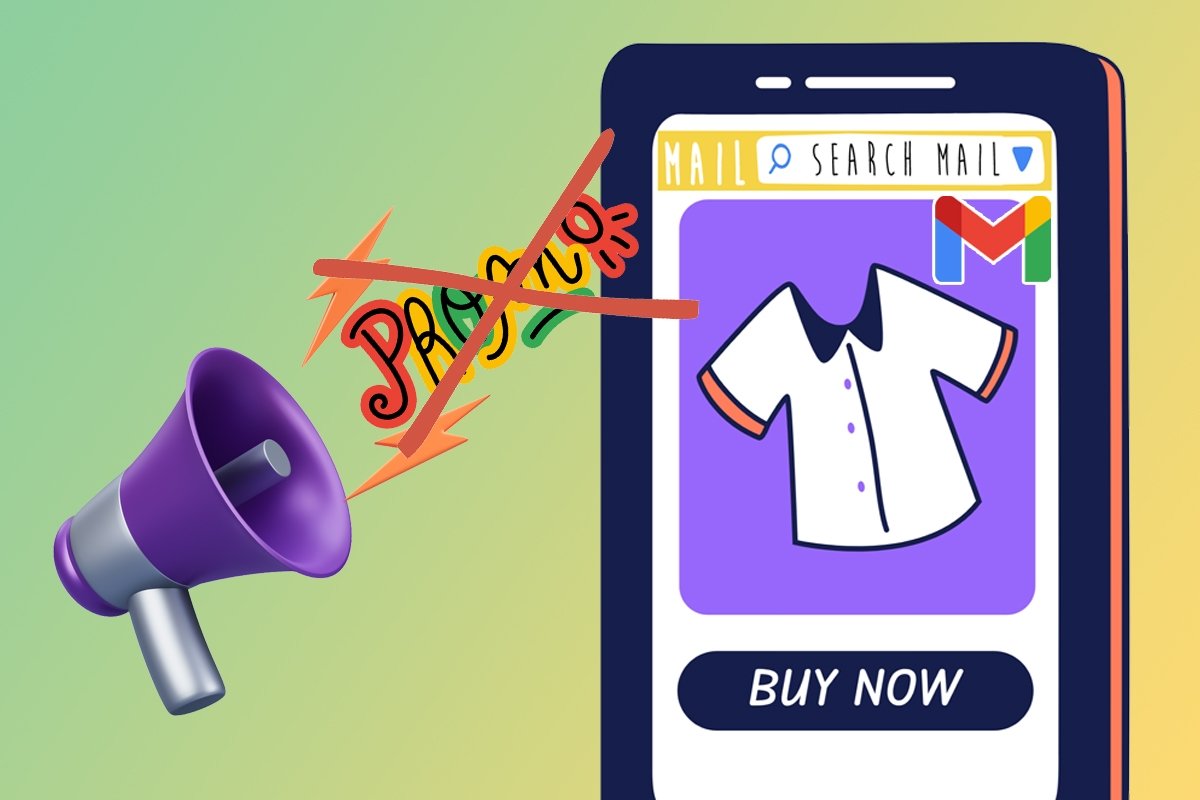The image depicts a screenshot captured from a cell phone, prominently displayed in the center of the frame, surrounded by a light gray background on all sides. At the top left corner of the screenshot, the time reads 6:38, while the upper right corner displays a Wi-Fi icon and a battery percentage indicator. The screen content is organized into five sections: "Primary" at the top, followed by "Social," "Promotions," "Updates," and finally "Forums" at the bottom.

A red diagonal arrow points downward towards the second check mark among four blue squares, each containing a check mark. The arrow specifically highlights the second square from the top. At the very bottom of the screen, the text "Starred Messages" appears in blue, followed by the phrase "Include in Primary, show all Starred Messages in Primary" written in gray. The entire content rests on a white background, with a small horizontal black bar positioned centrally at the bottom of the screenshot.